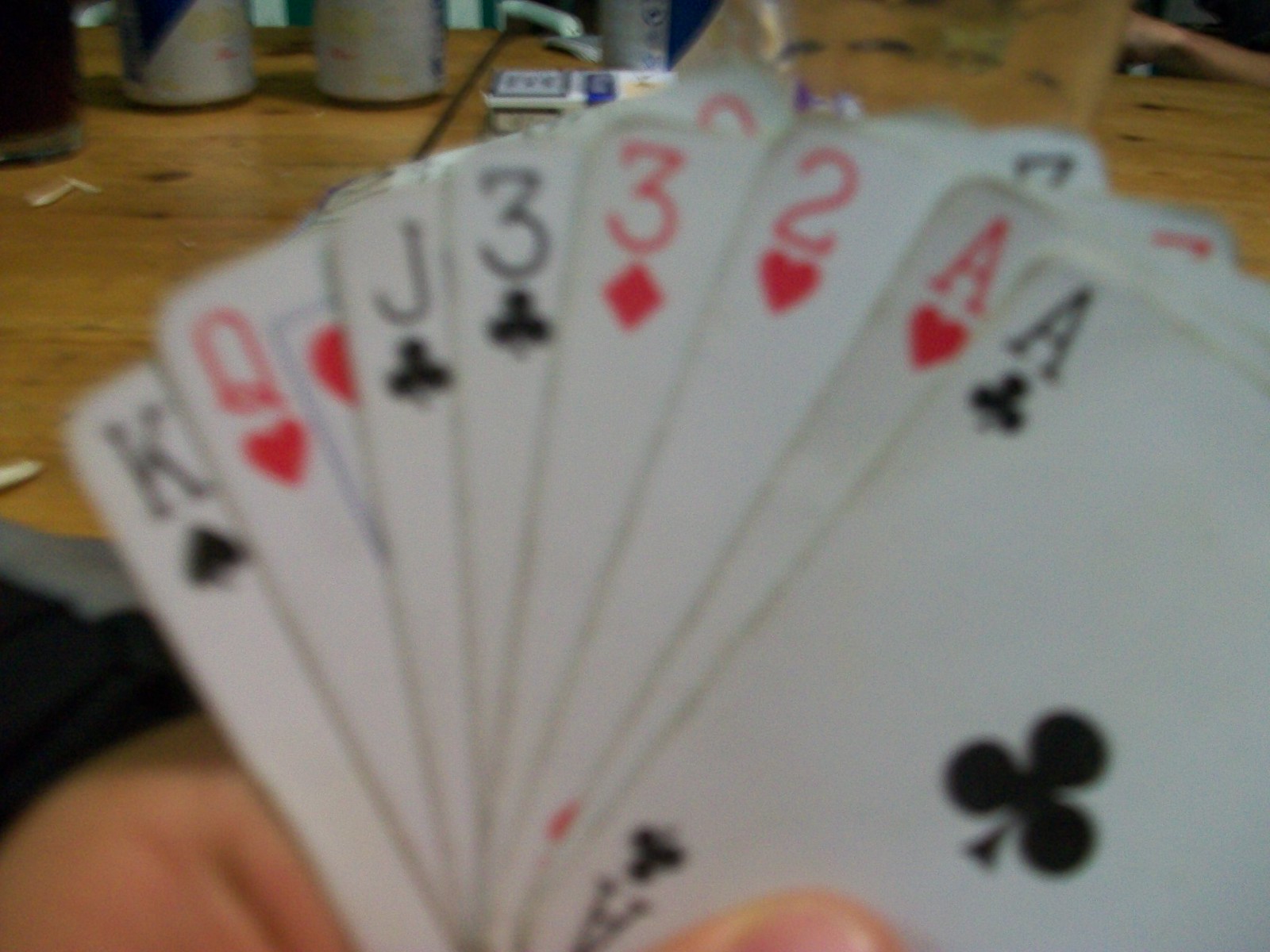In this blurred photograph, the main focus appears to be a fan of playing cards held by a person's hand, though the image clarity is low. The individual, who has fair skin, grips eight cards in a spread usually seen in poker. From left to right, the cards are the King of Spades, Queen of Hearts, Jack of Spades, Three of Spades, Three of Diamonds, Two of Hearts, Ace of Hearts, and Ace of Clubs. Each card is equally out of focus, adding to the challenging visibility. The background, albeit also blurry, reveals a wooden surface, possibly a table, along with some indistinct objects. Among these, two silver cans, a dark container, and several pieces of what seem to be white paper are distinguishable. There is also an unidentifiable item with a label, its text rendered unreadable by the blur. The positioning of the cards casts a shadow on the person's hand, suggesting the light source is situated behind them.